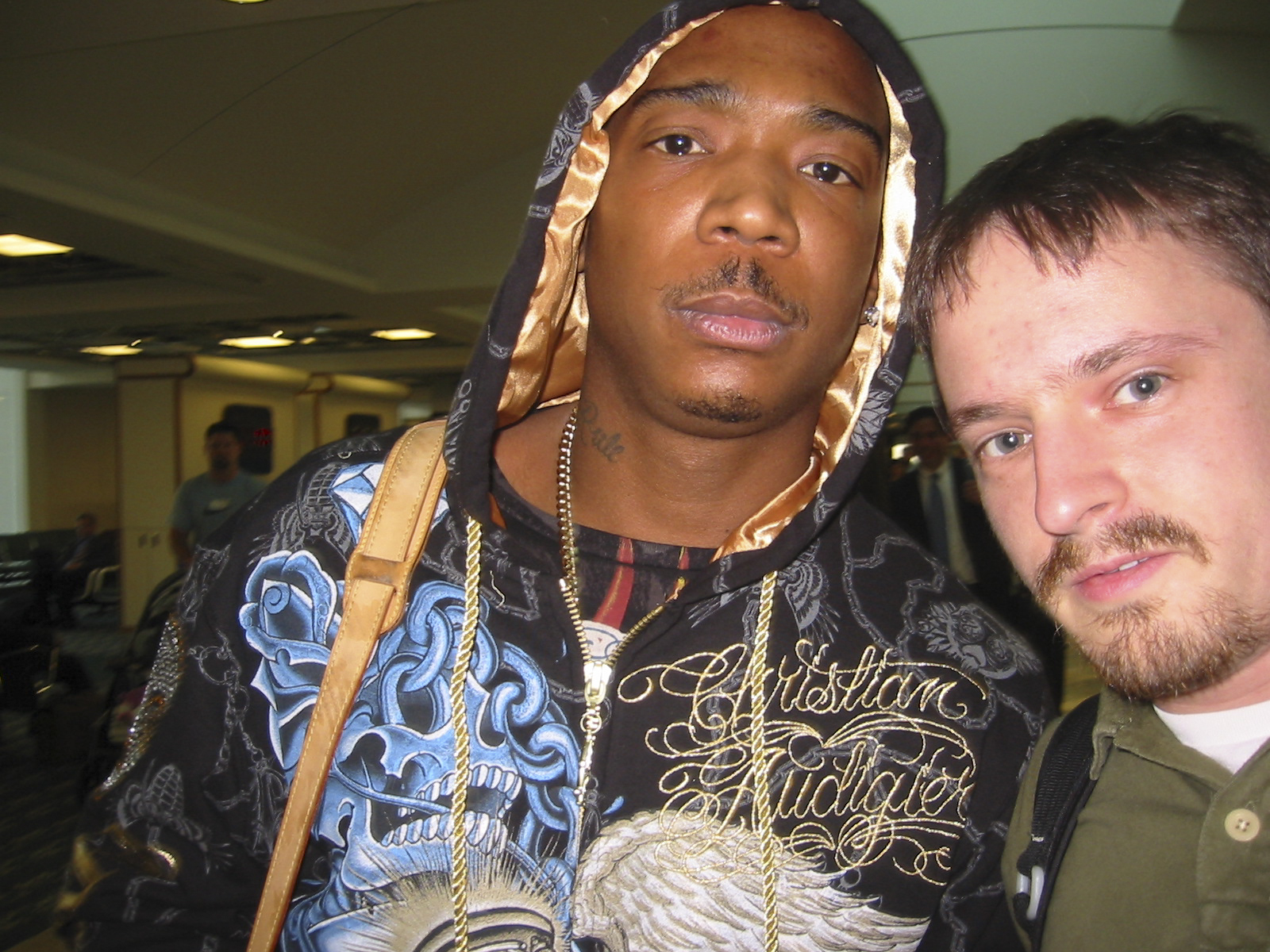The image depicts two men posing together, occupying the right side and center of the frame. The man on the left is an African-American, possibly a celebrity, dressed in a black hooded sweatshirt with a gold lining inside the hood. His sweatshirt features intricate details including a blue skull with chains on the right side of his chest, an abstract design with an angel wing, and cursive gold writing that is partially obscured. He's accessorized with multiple gold chains and has a tattoo on the right side of his neck. The man on the right is a white male with short brown hair, grey eyes, and a goatee. He is dressed in a green button-up polo shirt over a white t-shirt and has a black backpack indicated by the visible black strap. Both men are looking towards the camera, with neutral expressions. The setting appears to be an indoor space, possibly an airport or a hotel, characterized by blurred background figures and numerous seats.